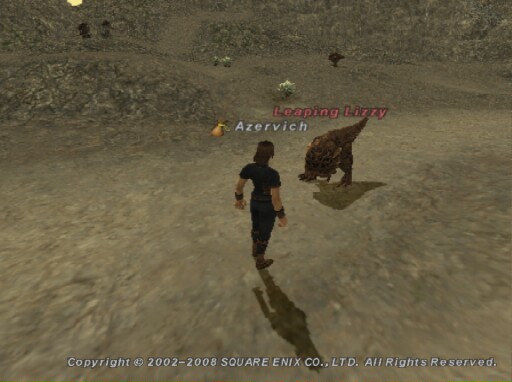This image appears to be a screenshot from an older video game, specifically from some time between 2002 and 2008, developed by Square Enix. The graphics suggest a 3D environment with a predominantly rocky, gray terrain, accented by patches of green plants hinting at a desert-like setting.

At the center of the image stands a character viewed from behind. This character is wearing a dark, short-sleeved shirt, matching dark pants, brown boots, and black wristbands on each arm. Their brown hair is visible, and a shadow extends behind them on the rocky surface. Above this character, white text spells out "Azervich".

To the right of the central character is a short, stocky creature resembling a dinosaur or an oversized lizard, characterized by a big head and a short tail. This creature is brown in color and labeled "Leaping Lizzie" in pink text above its head. 

At the bottom of the image, white text reads: "Copyright 2002-2008 Square Enix Company Ltd. All rights reserved."